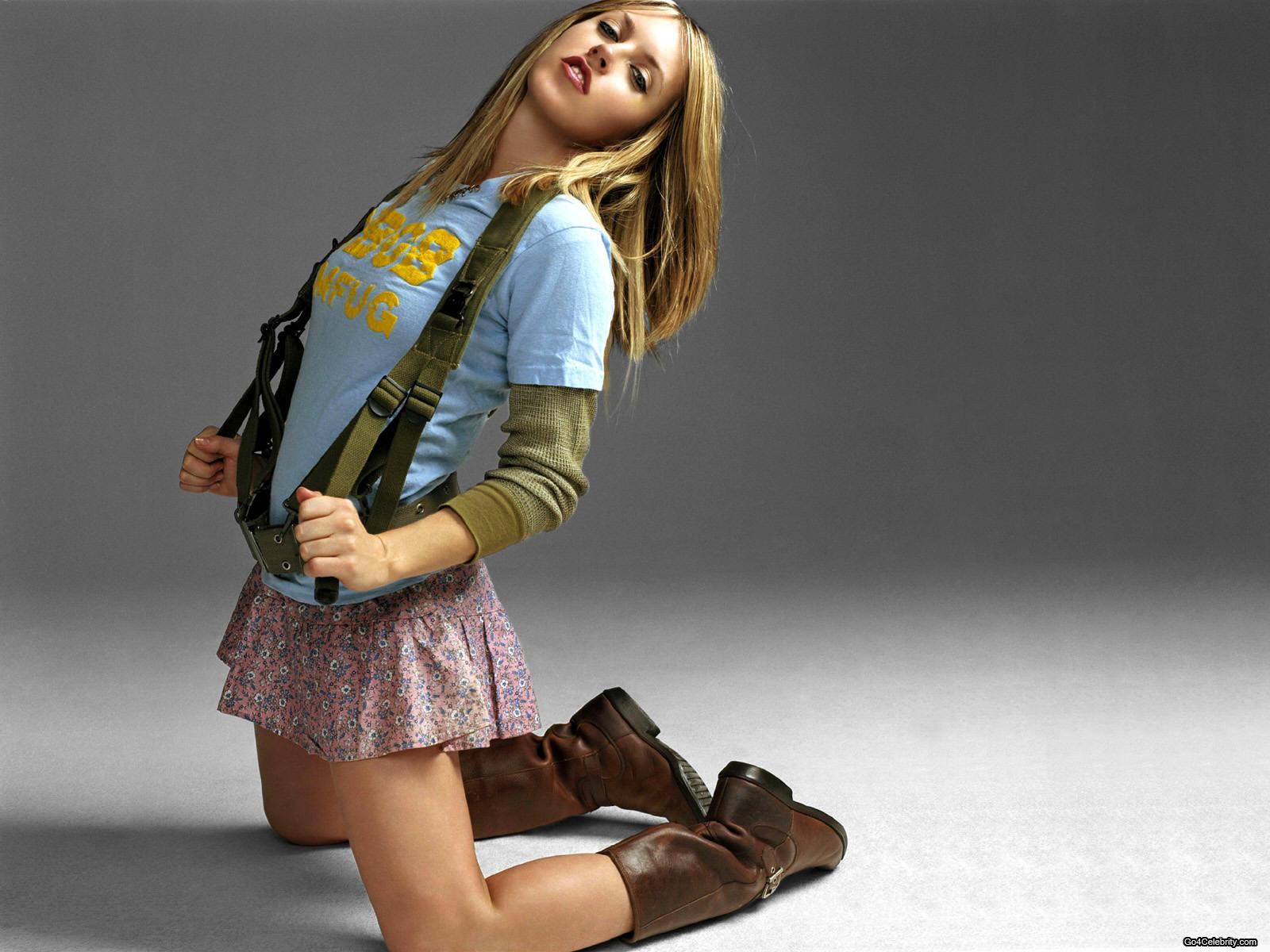The photograph features a young woman modeling in a studio setting with a seamless light gray floor curving up to a dark gray wall, giving an illusion of no distinct boundary between the two. Positioned more to the left side of the photograph, she is kneeling with her back arched, her head pointing towards the top right corner while her body faces the left. The woman, with her blonde hair falling below her shoulders, wears red lipstick and makeup around her eyes. Her attire consists of dark brown leather boots with silver buckles, a short pink skirt adorned with a white and purple floral pattern, a green long-sleeved shirt slightly rolled up, and a blue short-sleeved T-shirt featuring unreadable yellow text. Additionally, she is seen holding the straps of a green harness or possibly suspenders, adding a dynamic element to her pose.